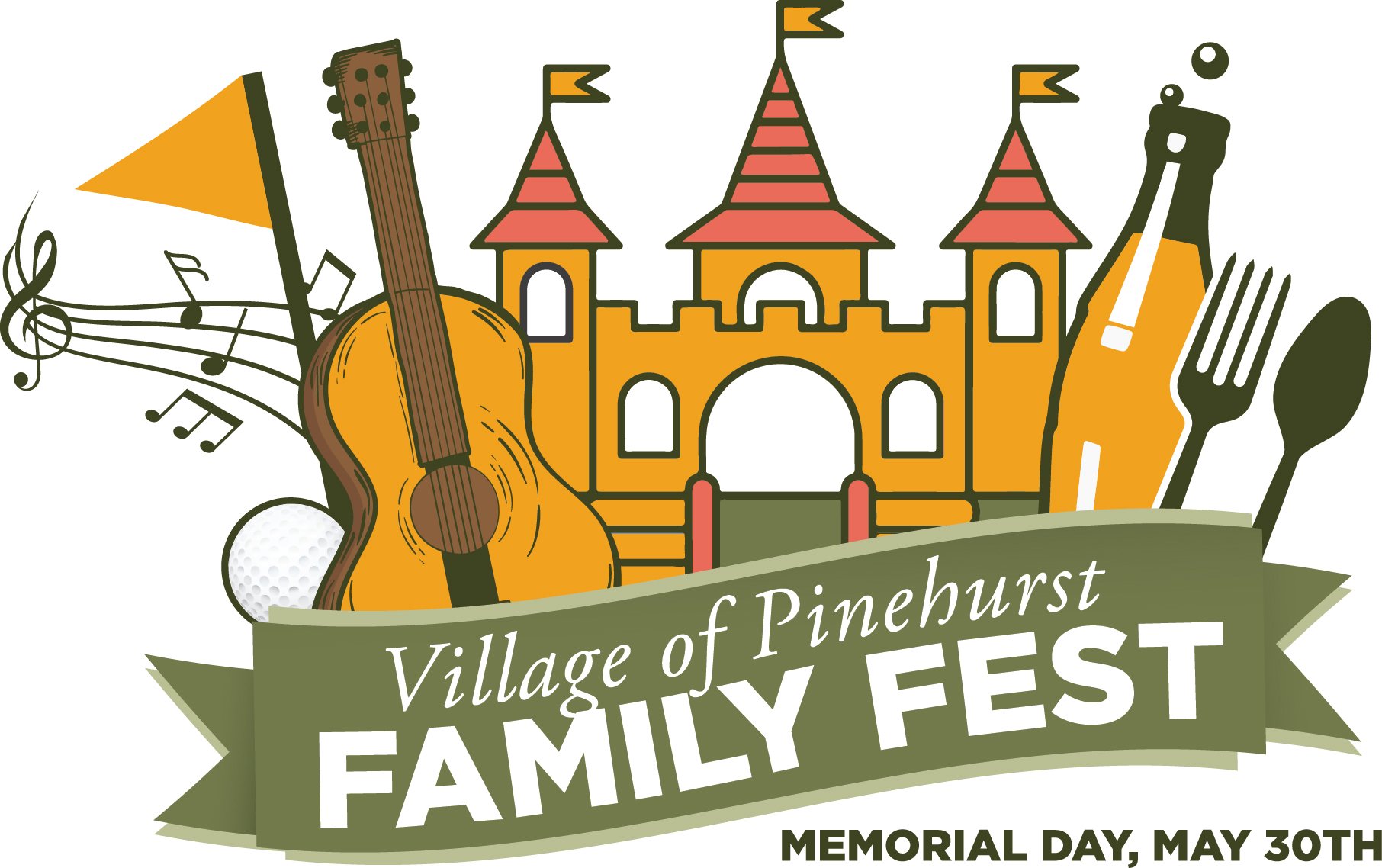This advertisement for the Village of Pinehurst Family Fest showcases a vibrant, cartoon-style design on a white background. Dominating the upper portion is a whimsical, yellow castle with three towers, each adorned with a red triangular roof, windows, and a flying yellow flag. Below the castle, extending across the bottom of the ad, is a green banner with elegant white lettering that reads "Village of Pinehurst Family Fest," with "Family Fest" in capital letters and "Village of Pinehurst" in a script font. Just beneath this banner, in bold text, it states "Memorial Day, May 30th."

On the right side of the castle, there is a vector art depiction of a bottle containing orange liquid with bubbles rising from the top, alongside a black fork and spoon. To the left of the castle, an orange acoustic guitar is displayed, with lively music notes emanating from it. Close by, a golf flagpole topped with a pointy triangular flag and a white golf ball adds to the festive atmosphere. The combination of these graphical elements creates a playful and engaging visual that highlights the various activities and attractions of the Family Fest.